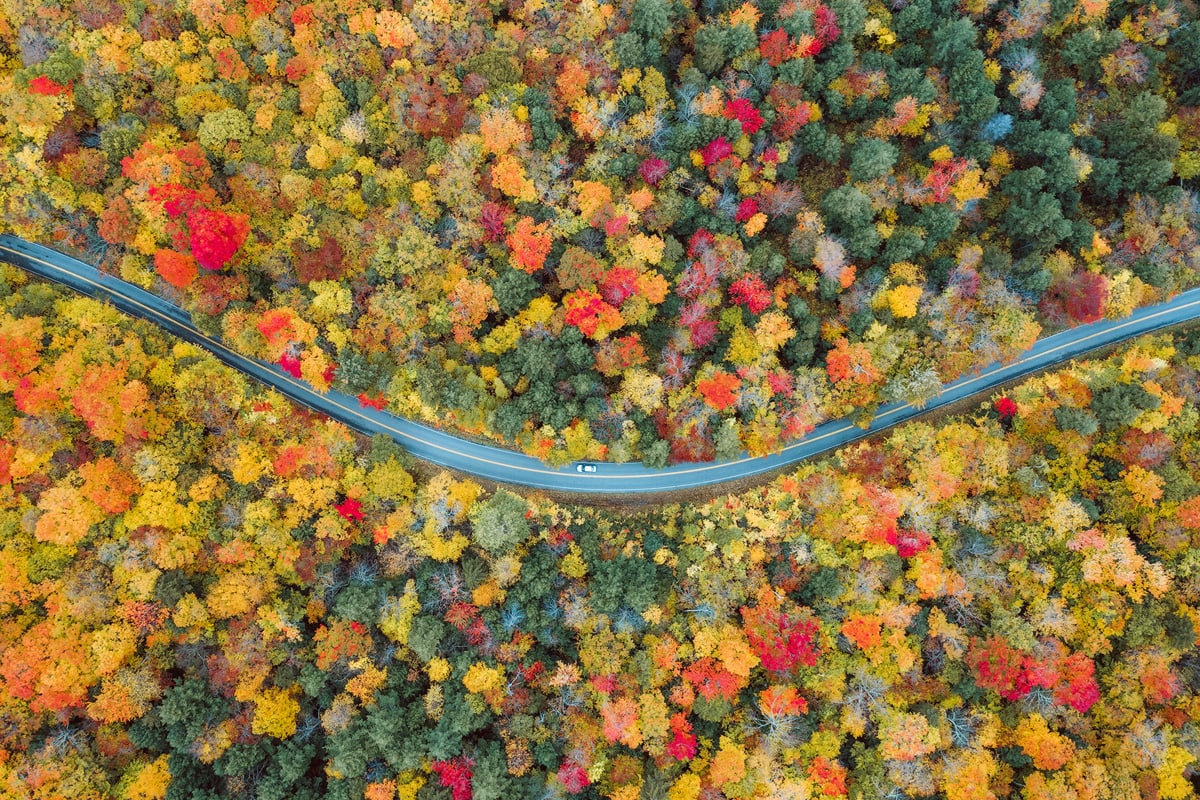An extreme aerial view shows a winding highway cutting through a vibrant forest bathed in the brilliant colors of fall. The road stretches from left to right, curving gently to form a slight smile-like shape. A solitary white vehicle, possibly an SUV, travels from right to left on the asphalt road marked by a solid yellow line. The forest surrounding the road is a spectacular tapestry of colors, featuring green pines, and foliage in shades of yellow, red, orange, blue, and purple, creating a striking, almost surreal landscape. This breathtaking scene, possibly captured by a drone, raises questions about its authenticity, yet it's a place that beckons to be visited.